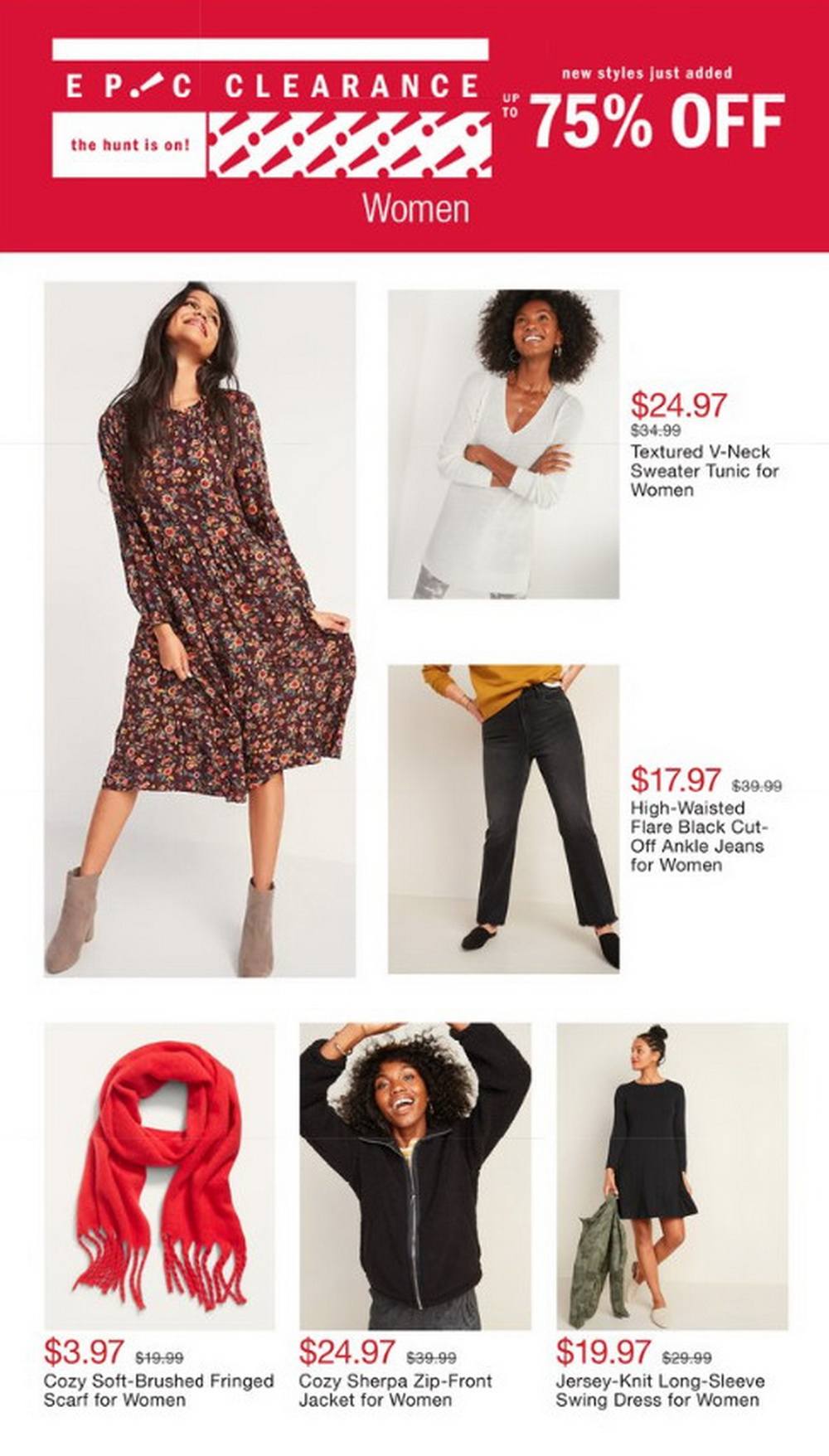This image is an advertisement for a clearance sale on women's clothing and accessories. The ad is designed with a prominent red banner that spans the top width, adorned with white text. On the left side of this banner, the phrase "Epic Clearance" is boldly displayed, with the letter "i" creatively slanted from bottom left to top right. Adjacent to this, it declares a massive "75% Off!" Below this, a smaller white bar emphasizes that "New Styles Just Added." At the bottom center of the red banner, the word "Women" is prominently featured.

Beneath the red banner, the background transitions to a clean white, organizing the content into six distinct squares. Dominating the left side is the largest square, showcasing a woman with sleek black hair wearing an elegant dress. To her right, another square features a woman adorned in a textured V-neck sweater, priced attractively at $24.97. This layout aims to capture the viewer's attention with its clear, visually appealing design, while highlighting the incredible deals available in this women’s fashion clearance event.